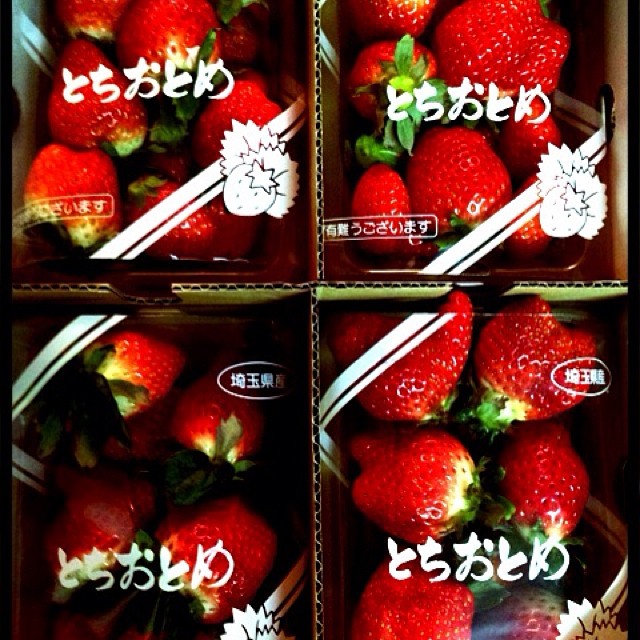This color photograph shows an aerial view of four neatly arranged boxes of strawberries. Each box, made from greenish-brown cardboard, contains approximately six to seven large, ripe, and bright red strawberries, each crowned with a small green stalk. The boxes are covered in clear cellophane, which bears white, non-English text, possibly in an Eastern script. The background of the image is a deep black, providing stark contrast to the vibrant strawberries. The lower left corner of each box features a diagonal white band with a drawn profile of a strawberry adorned with two large white leaves. Similarly, there is another white band along the upper left corner. On the right-hand side of this band, a small oval logo with unreadable text adds another visual element. The strawberries are tightly packed, with some overlapping each other, their stems either prominently displayed or hidden, contributing to the richness of the visual texture. The overall lighting from above accentuates the vivid colors and details, making the strawberries appear even more enticing and ready to eat.